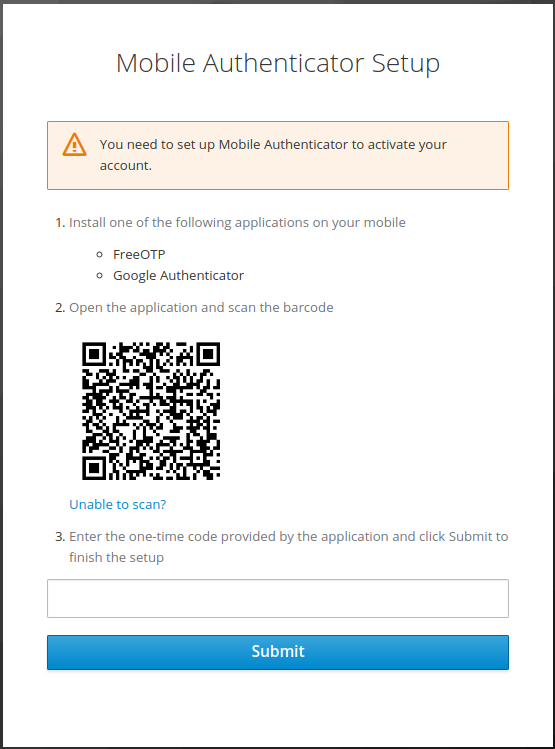The image depicts a vertical rectangle bordered in black with a white interior, serving as a mobile authenticator setup guide. At the top, the title "Mobile Authenticator Setup" is prominently displayed. Below this title, an orange box with an orange outline contains an orange triangle marked with an exclamation point. Inside this box, a warning message reads: "You need to set up a mobile authenticator to activate your account."

The instructions follow in a detailed step-by-step format:
1. "Install one of the following applications on your mobile device," with bullet points listing "FreeOTP" and "Google Authenticator."
2. "Open the application and scan the barcode." Below this sentence is a note in blue text: "Unable to scan?" indicating an alternative method is available if scanning the QR code is problematic.
3. "Enter the one-time code provided by the application and click Submit to finish the setup."

A gray-bordered data entry field is provided where users can input the one-time code. Below this field is a blue button of the same size as the data field, featuring the word "Submit" in white text. 

The color scheme includes black, white, light orange, dark orange, gray, and blue. The instructions are clear, providing users with a straightforward way to set up their mobile authenticator, though the image confusingly refers to a QR code as a barcode.